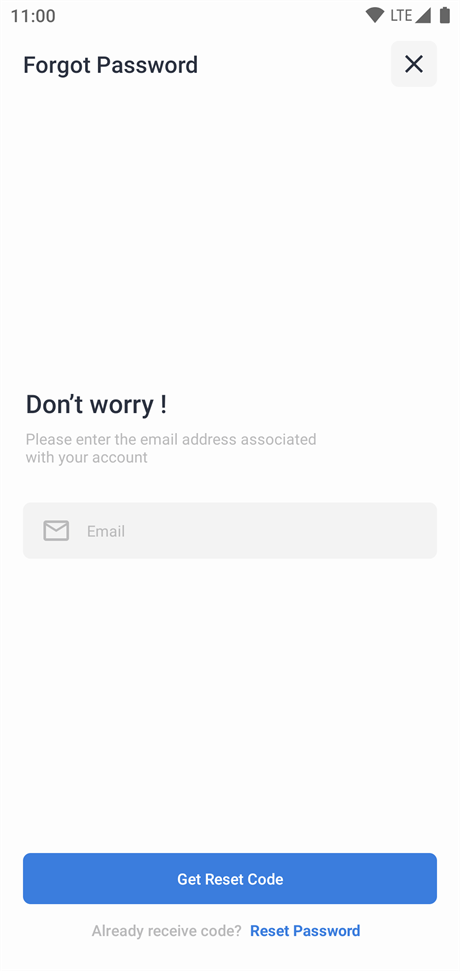The image is a screenshot taken from a phone at 11 o'clock. At the top of the screen, it displays the text "Forgot Password" followed by an "X" button option for closing the page. Centrally located on the screen are the reassuring words, "Don't worry. Please enter the email address associated with your account." Below this prompt is a blank email input field for the user's email address. Toward the bottom of the page, there is a prominent rectangular blue button labeled "Get Reset Code" in white font. Beneath this button, the caption reads, "Already received code? Reset Password." This text provides an alternative action for users who already have a reset code. Finally, for additional information, it directs viewers to visit www.fema.gov.